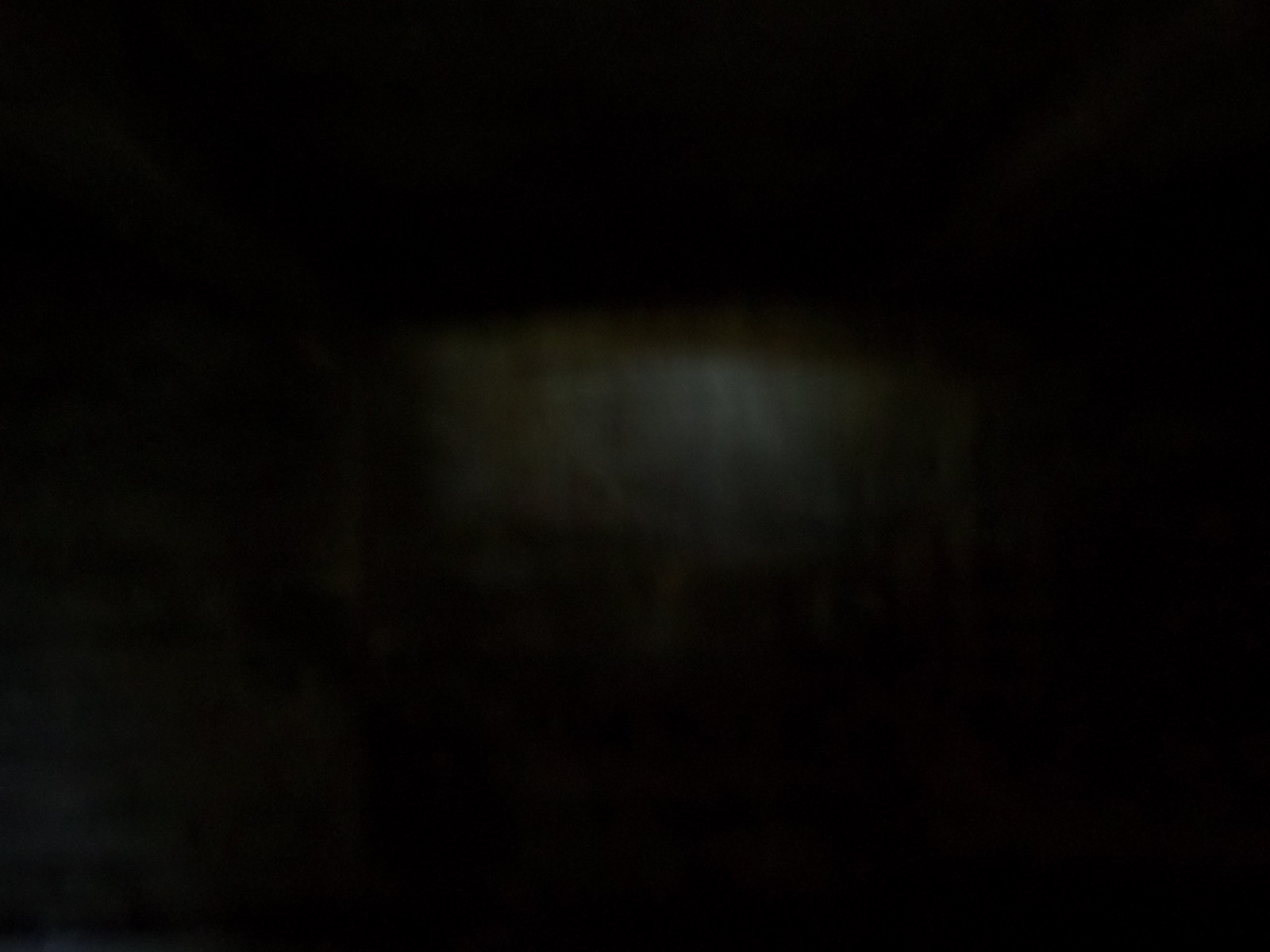The image presents a predominantly black background with minimal visible elements. In the center, there is an indistinct, lighter rectangular area with hints of green around its edges and a light blue hue within. This central figure is devoid of clear definition and appears out of focus, resembling a whitish, greenish-brown mist. Additionally, the lower left-hand corner features a slightly lighter section with what appears to be a dark green square and a touch of lighter blue, separated by a faint line. The image appears to have been taken at night or in very low lighting conditions, lacking any discernible details, text, or describable features, and the highlighted sections occupy less than 10% of the entire composition.